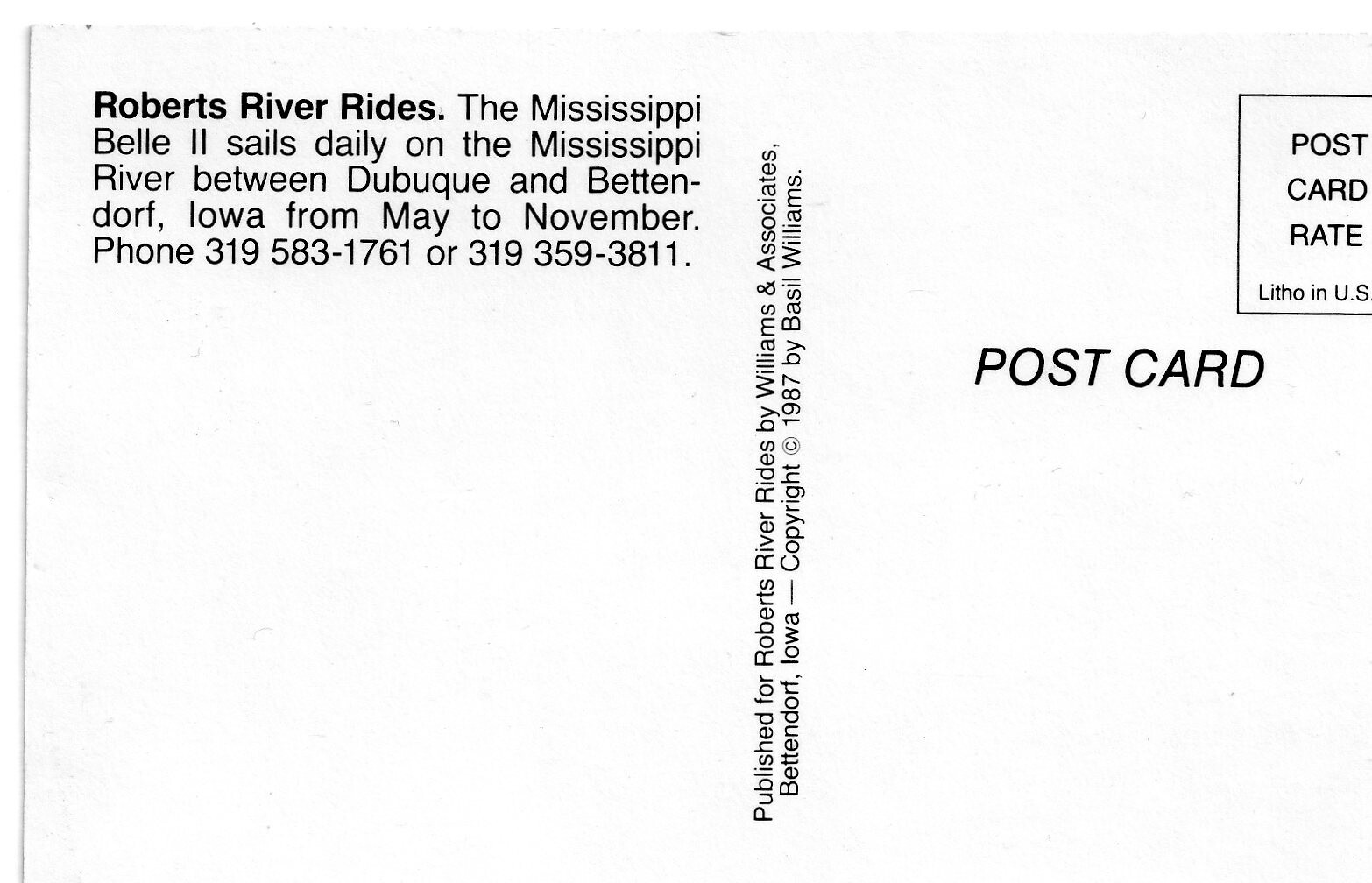This is an image of the back of a postcard, showcasing a straightforward black and white design. On the left side in bold text, it reads: "Roberts River Rides, the Mississippi Belle II sails daily on the Mississippi River between Dubuque and Bettendorf, Iowa from May to November. Phone 319-583-1761 or 319-359-3811." At the top right corner, there is a square where stamps are designated, marked with the text "Postcard Rate, Litho in U.S." Below this square, the word "Postcard" is clearly printed. Centrally placed and turned 90 degrees, the text states: "Published for Roberts River Rides by Williams and Associates, Bettendorf, Iowa. Copyright 1987 by Basil Williams." The overall layout is clean and minimalistic, emphasizing the essential information about the Roberts River Rides and its publishing details.